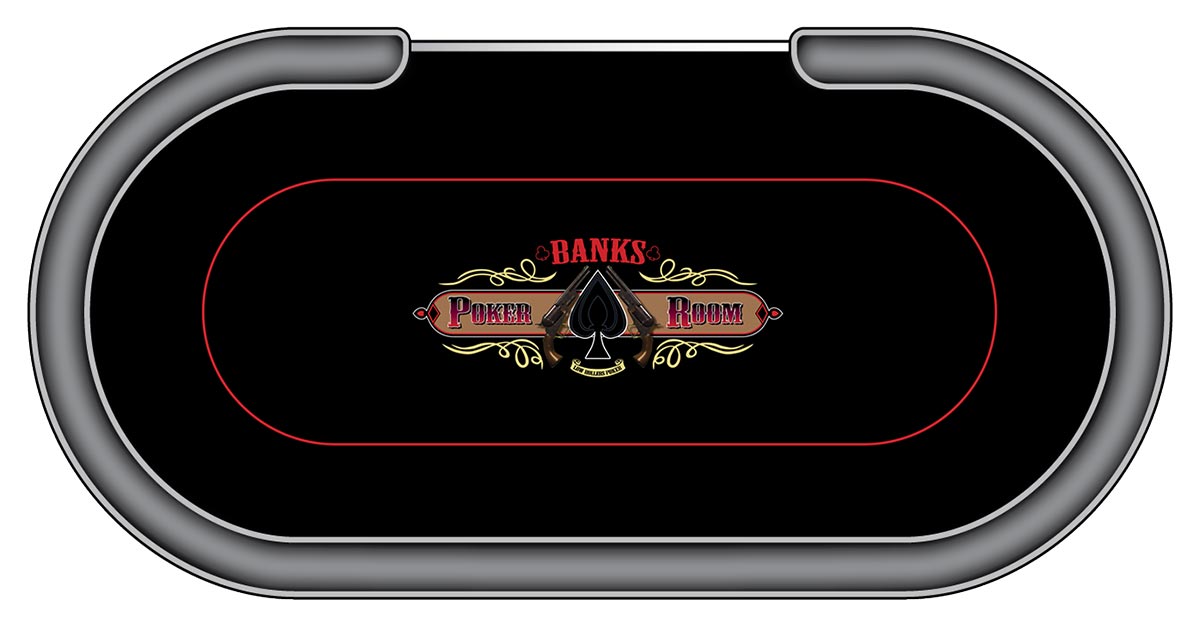The image is a computer-generated, top-down view of an oval-shaped poker table with a gray, padded border that almost encircles the entire table but leaves an open spot at the top for the dealer. The table surface is black with a red oval in the center that features the text "Banks Poker Room" in red letters. Within this red oval, there is a spade symbol reminiscent of a playing card, flanked by two revolvers with wooden handles pointing upwards. The background of the poker table appears to be made of a wooden material, enhancing the detailed, realistic look of the graphic.